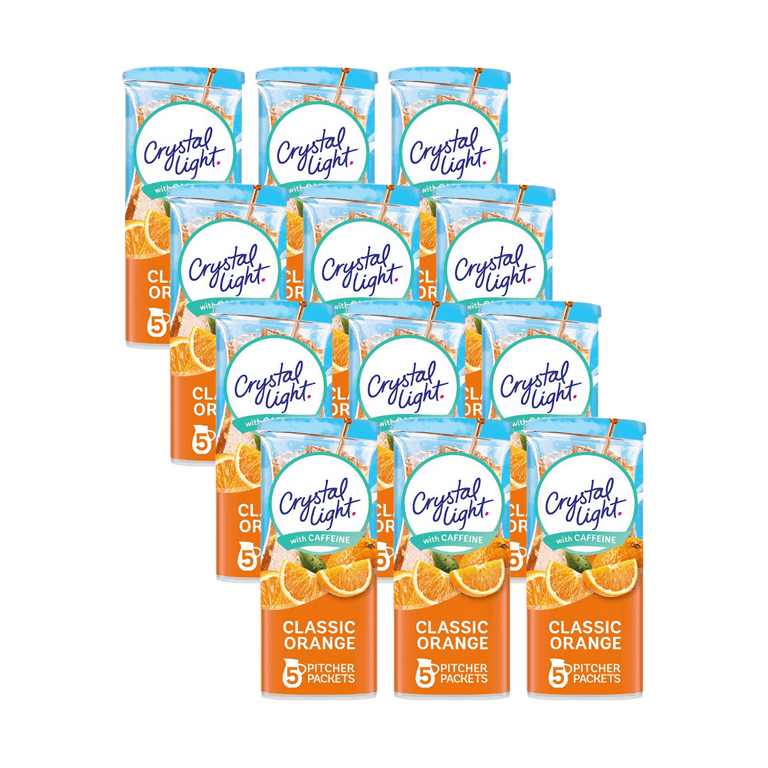The image is a color photograph in portrait orientation, showcasing four rows of Crystal Light orange drink mix packages, with three identical packages in each row, organized on a diagonal from top left to bottom right. The background is white, having been photoshopped out. Each package features a round white circle with an aqua border at the top, inside of which “Crystal Light” is written in dark blue script. Below this, an aqua banner with white text states "with caffeine." Below the banner, there are vibrant slices of orange, and under that, the words “classic orange” are displayed in white font against an orange background. In the bottom left corner, a white gallon pitcher icon with an orange number "5" is depicted, accompanied by the text "pitcher packets" in smaller white font to its right. The image employs a photographic representational realism style.